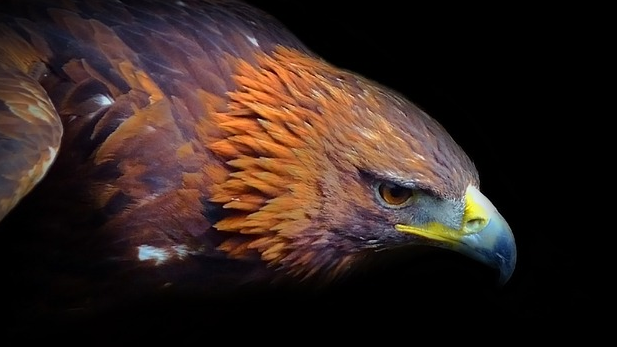This close-up photograph captures a striking side profile of an eagle, showcasing the majestic bird's face, head, and a portion of its upper body. The eagle is oriented towards the right, and its plumage exhibits a unique blend of orange and purple hues. The prominent beak of the eagle is primarily blue, featuring a yellow section near the base and a dark blue tip. The eagle's piercing brown eyes convey a determined expression. The background of the image is completely black, which further accentuates the vivid colors and formidable presence of the eagle.